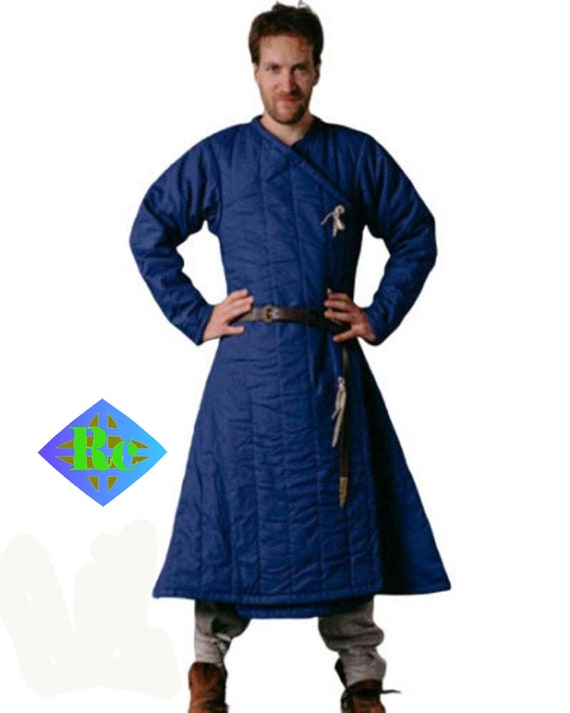In this photograph, a young Caucasian man, likely in his 30s, stands confidently against a white background with a slight smile. He is wearing a detailed costume that includes brown leather boots and beige or light-colored pants. His striking attire features a long, crisscrossed quilted blue overcoat that extends past his knees, fastened with a brown belt and leather strap. The overcoat has long sleeves and appears to be part of a traditional or fantasy-inspired outfit, possibly indicating a ninja theme or a historical robe. He is standing with his hands on his hips, showcasing his ensemble proudly. The man also has short brown hair and a light beard. To the left of him, there is a blue diamond-shaped graphic with the letters "R" and a smaller "c" in the center, adding a modern or branded element to the image.